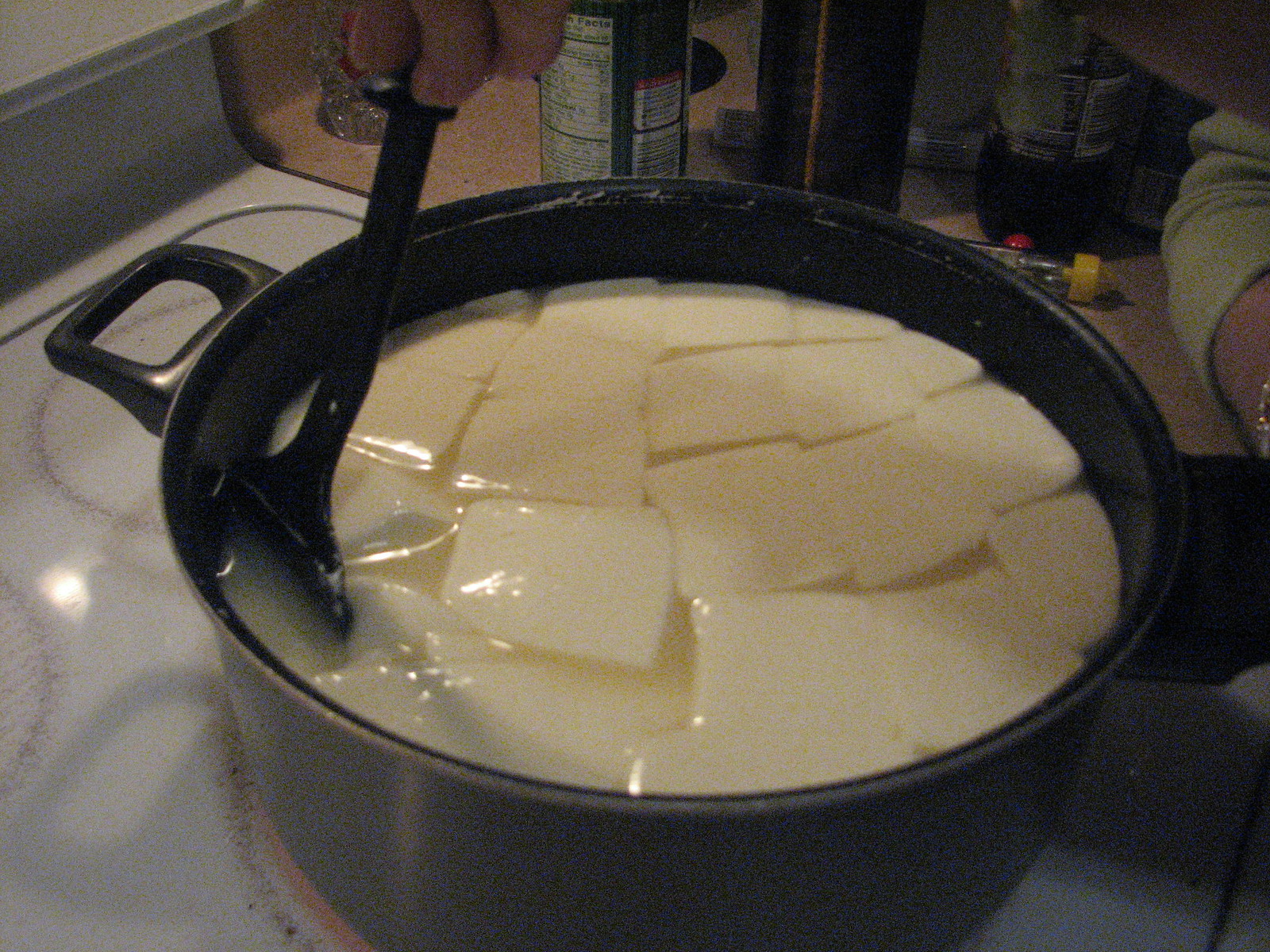A detailed indoor kitchen scene features a black pot on a white four-burner stove. The pot is filled nearly to the brim with a liquid and numerous small, white, square-shaped items that resemble cheese curds or gel-like cubes. A hand, seen from the fingertips, holds a black spatula, actively stirring the pot. Above the pot, the kitchen setting includes a visible wooden countertop adorned with several containers, one of which prominently displays a nutrition facts label. The presence of a table is suggested in the background, along with cans that could possibly contain beer or other beverages. The overall focus is a close-up of the cooking process, emphasizing the interaction with the utensil and the intriguing contents of the pot.